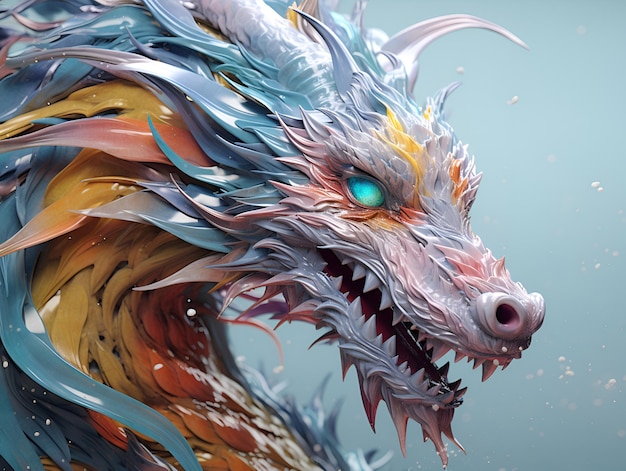The image depicts a vividly colored, artistically rendered dragon with a striking, detailed appearance. Set against a bright blue, gradient background sprinkled with white flecks, the dragon's head and neck exhibit a flowing, dynamic fur texture. The dragon's snout is a blend of whitish-pink hues with yellow and orange highlights, transitioning into teals, blues, greens, and rosy oranges towards the back of its head. Its striking, gradient-filled eyes lack pupils and transition from light green to an aqua blue-green, exuding a fierce, intense expression. The dragon's mouth is partly open, revealing sharp, white, dog-like teeth, complemented by large nostrils and a vividly colored, intricately detailed fur pattern spanning whites, pinks, purples, yellows, and oranges.